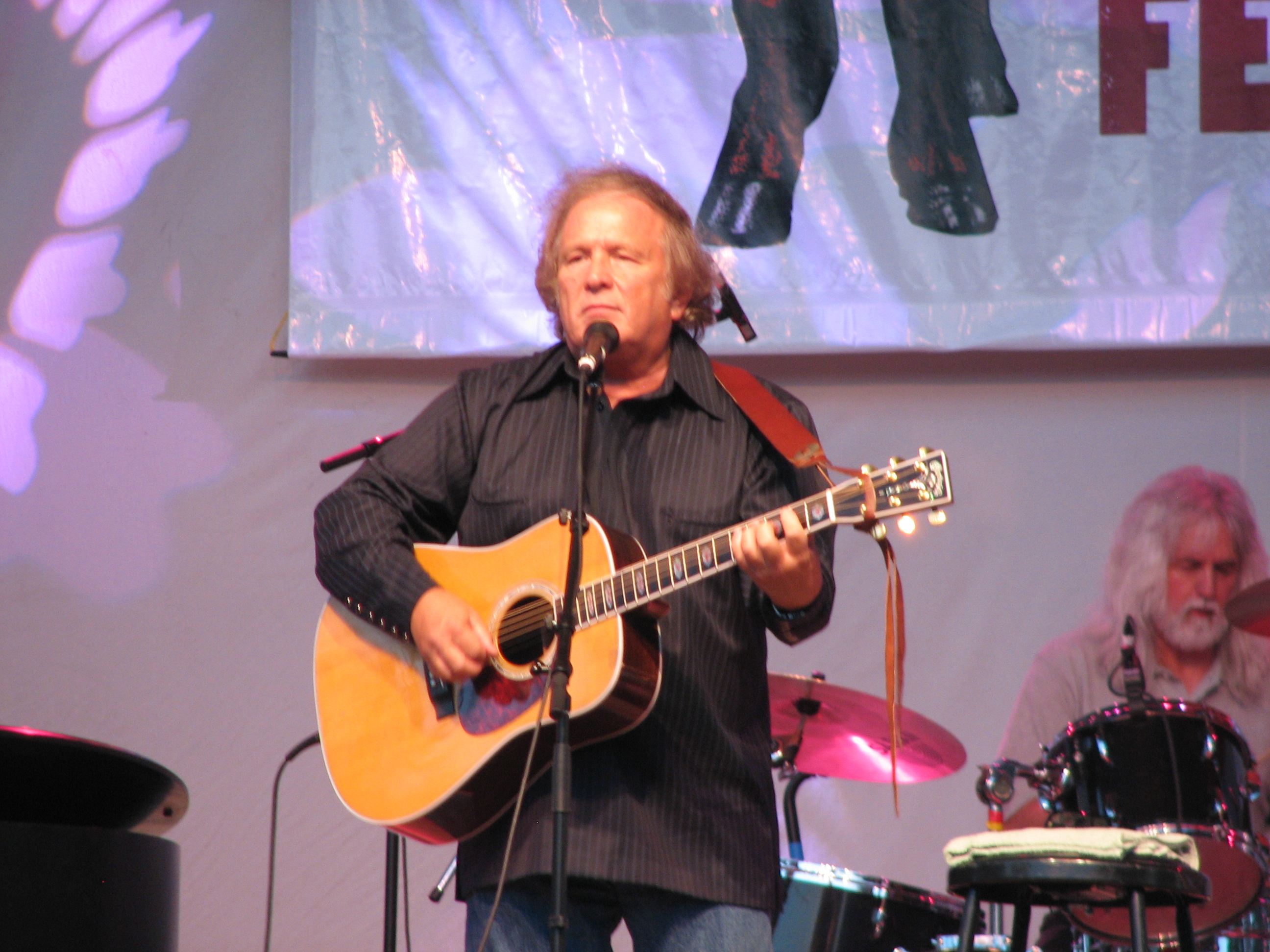The image captures a live stage performance featuring two older male musicians. The foreground focuses on a man approximately 60 years old with thinning, combed-over hair. He is dressed in a black, pinstripe, long-sleeve shirt and blue jeans. He stands center stage, strumming an acoustic guitar hooked up to a speaker via a cord. Positioned behind him is a drummer with long, silver hair and a matching beard, playing a black drum set with a cymbal. Both men have a scruffy appearance. The backdrop is a grayish-white wall with shadows cast by stage lights. To the upper right, a partially visible plastic banner hangs, displaying black hooves and partial letters "F" and "E" in black and red.